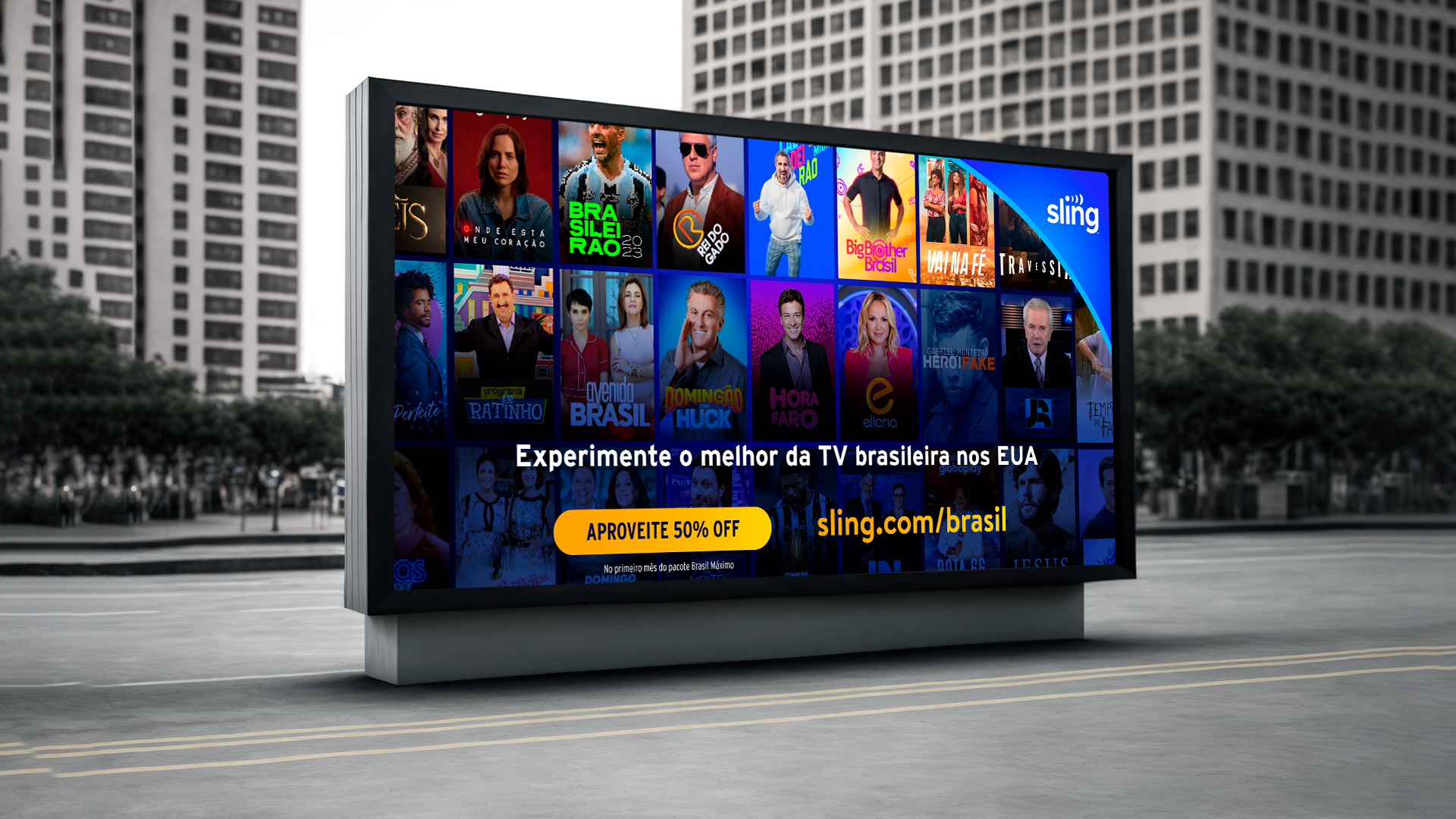The photograph captures a bustling urban scene featuring a prominent digital billboard set against a monochromatic background. In the foreground, a gray street marked with three yellow lines spans from left to right. Dominating the center of the image is a large, rectangular digital display mounted on a gray, stone-like base that somewhat resembles a TV screen. This digital billboard displays a colorful advertisement for Sling TV, prominently featuring the Sling logo in the upper right corner and the text "Sling Brazil" along with a "50% off" promotion and a website link to "sling.com/brazil" toward the bottom. The screen showcases a variety of streaming TV show icons, represented by small rectangular posters with celebrity images and show titles.

The street is bordered by a row of tall trees, creating a natural separation from the city's backdrop. Flanking the billboard and trees are two tall, similar-looking buildings with multiple floors and windows, which appear dark gray in contrast to the vibrant billboard. The sky, visible between the buildings and above the trees, is a stark white, accentuating the grayscale environment and highlighting the colorful content on the digital display. These elements together create a vivid focal point on the billboard amidst the grayscale cityscape.